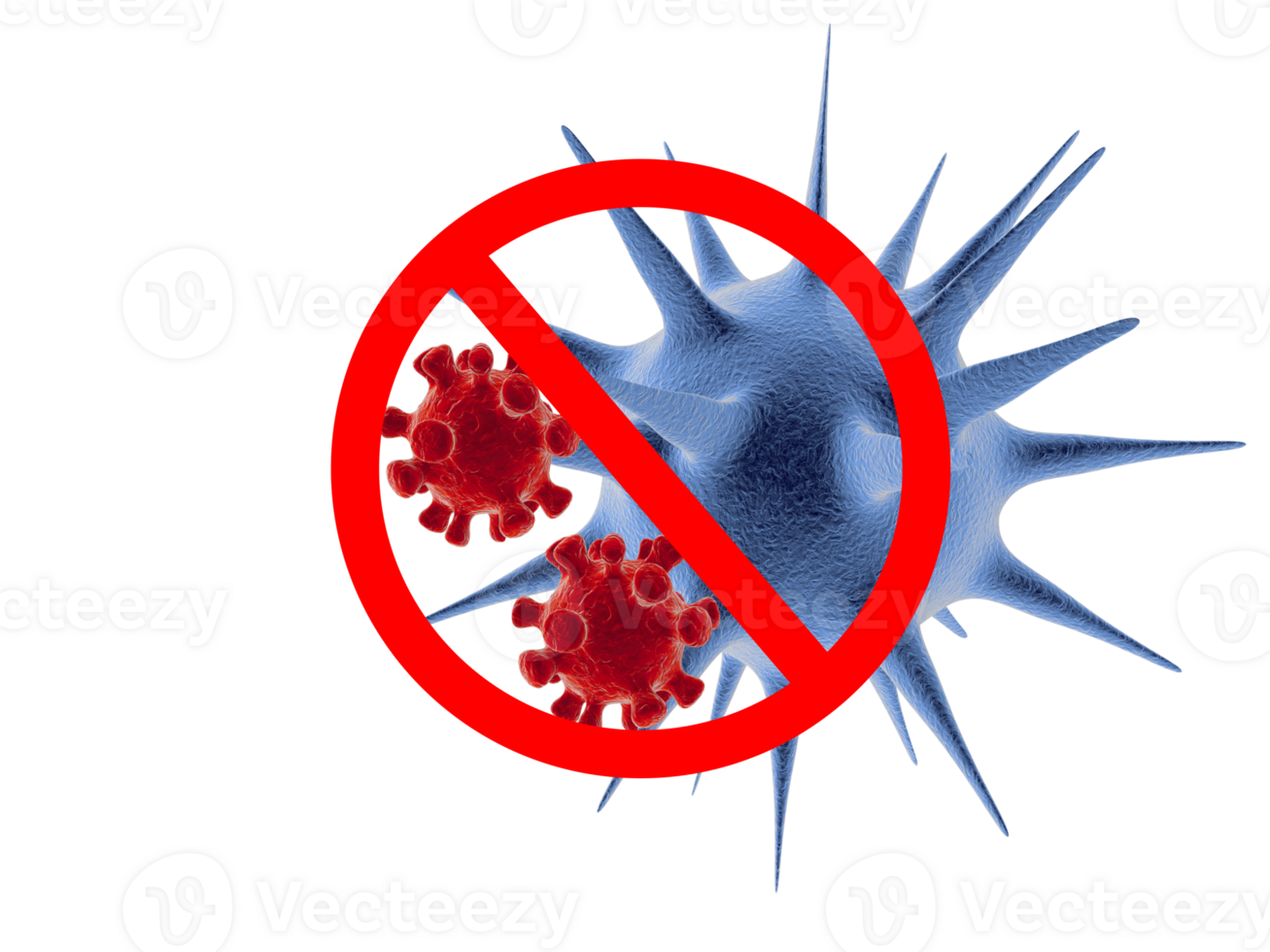This digital rendering depicts a virus or microbial structure against a predominantly white background, which is subtly overlaid with a watermark featuring a cursive "V" logo and the text "Vecteezy." The centerpiece of the image is a large, blue-toned, spiked sphere with varying spike heights and a raised, bumpy texture, suggesting a virus or a disease agent. To its immediate left are two smaller red spheres, each adorned with conical spikes that have bulbous ends, resembling suction cups or short protrusions. These red spheres also share the raised, bumpy texture found on the blue sphere and exhibit subtle darker red variations. Positioned above and slightly to the left, a prominent red circle with a diagonal line through it indicates a warning or prohibition, possibly symbolizing the containment or eradication of these depicted elements. The rendering is detailed with a slight presence of dark brown in the blue structure’s core, enhancing the depth and realism of the image.